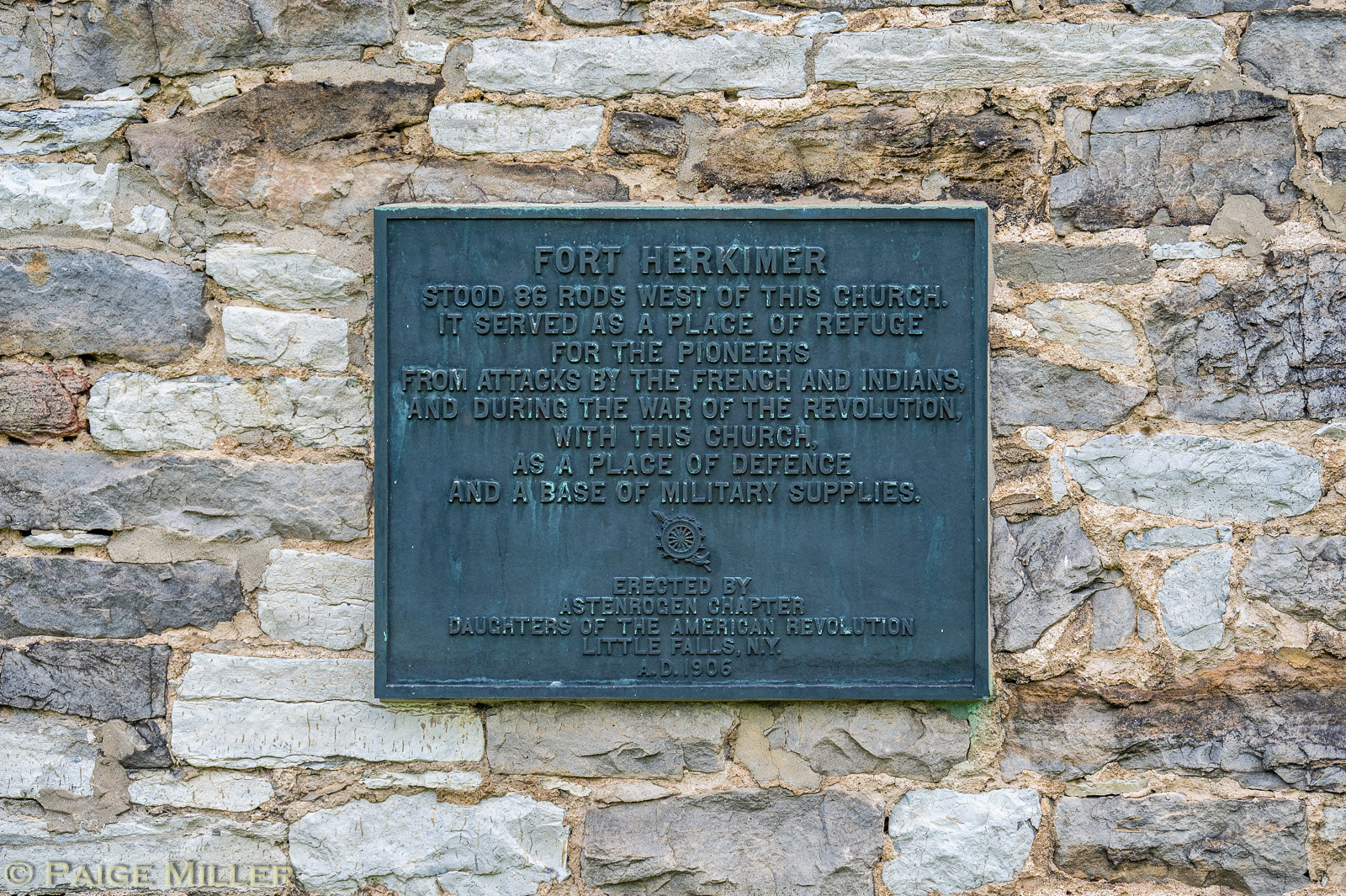The image depicts an outdoor scene showcasing a stone brick wall composed of various shades of gray stones interspersed with tan or orangey grout. Dominating the center of the wall is an aged, oxidized brass plaque that has turned a deep green color. The plaque details historical information, reading, "Fort Herkimer stood 86 rods west of this church. It served as a place of refuge for the pioneers from attacks by the French and Indians and during the War of the Revolution, with this church as a place of defense and a base of military supplies." Beneath this, there is a badge or seal resembling a compass, followed by an inscription that states, "Erected by Aston Rogan Chapter, Daughters of the American Revolution, Little Falls, NY, A.D. 1906." In the bottom left-hand corner of the image, there is a copyright watermark that reads, "© Paige Miller."